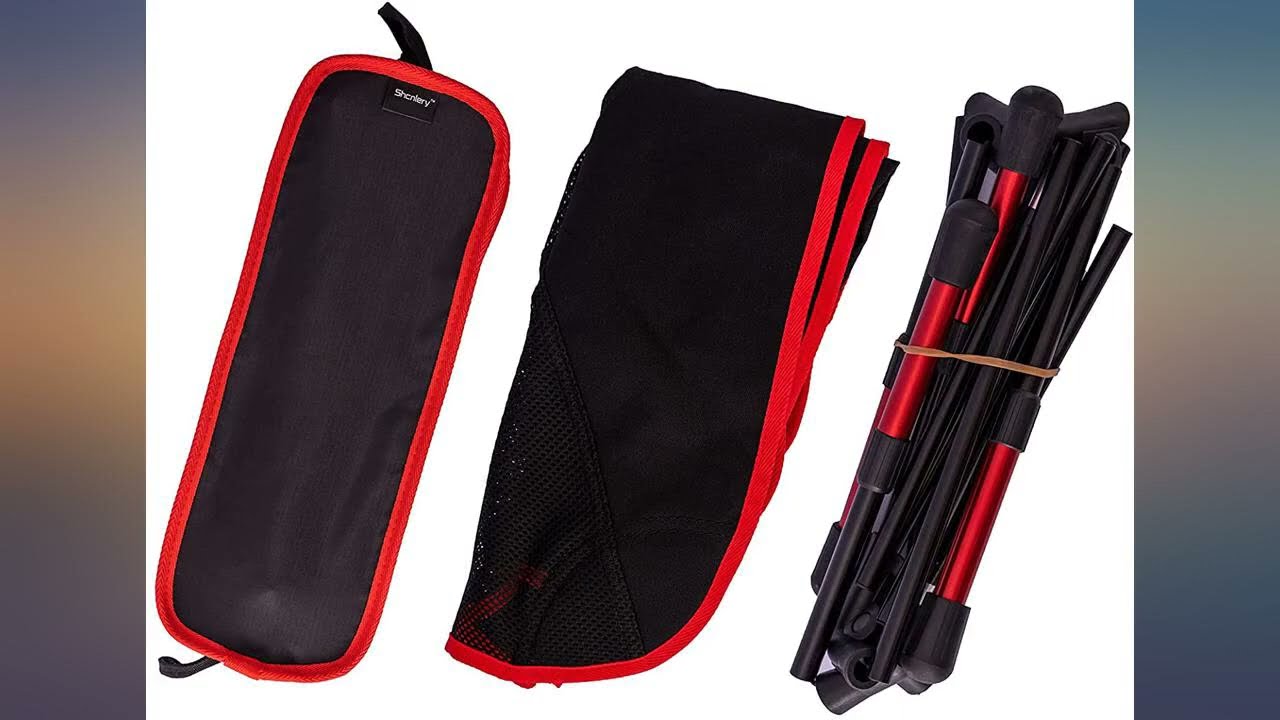The image features a compact and packable object with three distinct components, set against a plain white background. On the left, there is a black fabric carrying case with a red border, equipped with two straps and a rectangle label that reads "SHENLERY." In the center, a folded black mesh netting with a red border is displayed. To the right, an arrangement of interconnected red and black metal tubes, each capped with rubber ends, forms a base structure. The image is framed vertically on both sides: the left border transitions from dark gray to orange and back, while the right border shifts from bluish-green to yellow and orange before returning to bluish-green and gray. Together, these components suggest a foldable and portable lounge chair, designed for easy transport and assembly.